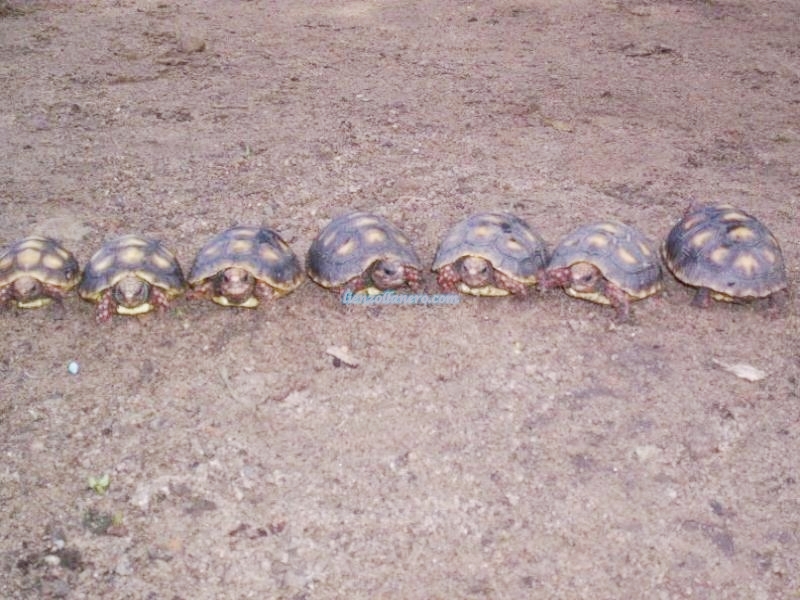In this bright afternoon photograph taken outdoors, a row of seven turtles is lined up on a sandy, brown dirt field that stretches from the left to the right side of the image. Each turtle is standing on bare ground scattered with small rocks and leaves, and a tiny piece of green plant is visible at the bottom left corner. The turtles, all with identical brown shells adorned with yellow spots, appear to be either preparing for a race or have been arranged for a photo. While the first six turtles are facing directly towards the camera, the seventh turtle on the far right is facing backwards. In the center of the image, a watermark reads "genzolanero.com" or "honzoffaner.com," subtly overlaying the scene.